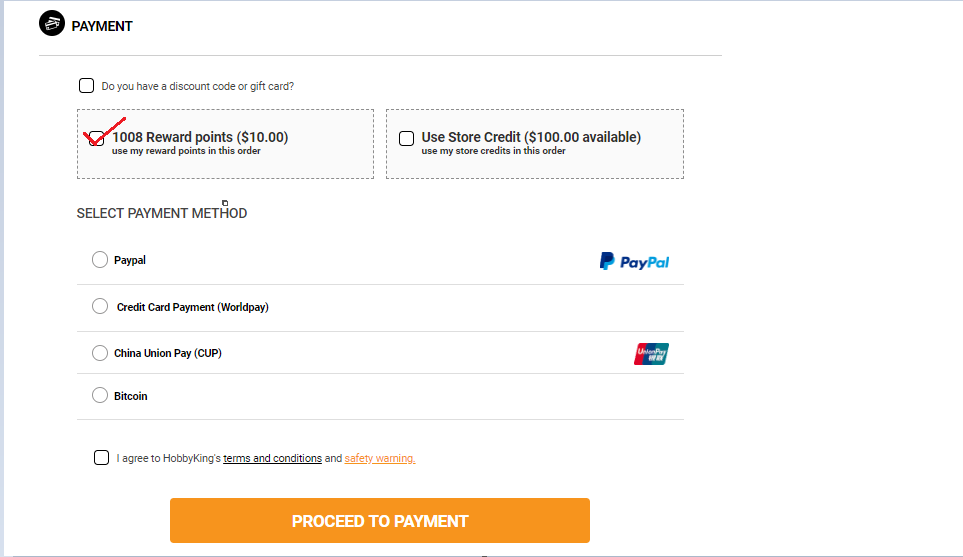This image appears to be a detailed screenshot of a payment page on a website. The interface is displayed within a horizontal, white rectangle that lacks a right-side border, and the remaining three sides are outlined with a gray line. In the top left corner, a black circle encloses a symbol that resembles credit cards, accompanied by the word “Payment.”

Below this header, there's a section inviting users to enter a discount code or gift card, with a checked box indicating that a discount or gift card has been applied. This area also displays text reading “1008 Reward Points ($10)” alongside an option to use reward points for the order, which has been selected.

Underneath, the page prompts users to select a payment method, offering various options indicated by clickable dots. The available methods are listed sequentially: PayPal, Credit Card Payment (WorldPay), China UnionPay (CUP), and Bitcoin.

Further down, there's a checkbox for users to agree to Hobby King's terms and conditions, as well as a safety warning. The page concludes with a large, prominent orange rectangle at the bottom, emblazoned with the words “Proceed to Payment” in white text, serving as the call-to-action button for finalizing the payment process.